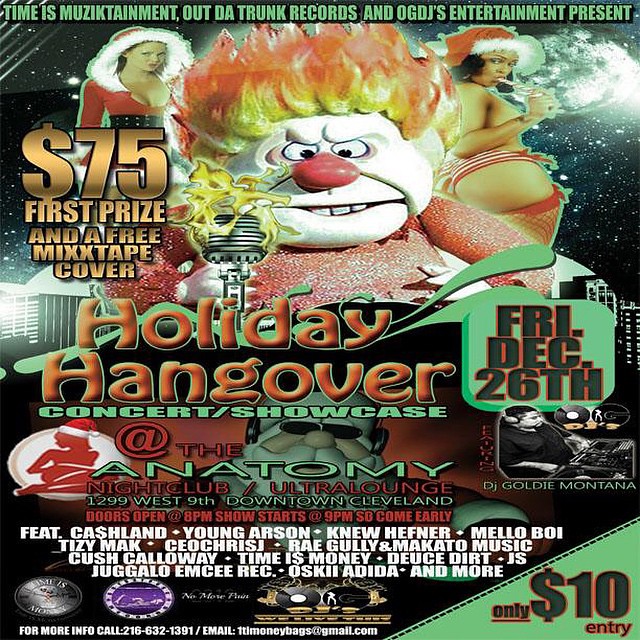A vibrant poster board announces an event with a chaotic blend of colors and images. At the top, it reads "Time is Musictainment Outta Trunk Records and OG DJs Entertainment present" in black and green writing. Dominating the center is an image of an enraged snowman with fire erupting from his head and a microphone. Flanking him are scantily clad women in snowman hats. Below this image, the poster states "$75 first prize and a free mixtape cover," alongside details of the event: "Holiday Hangover, Friday, December 26, $10 entry fee." The event, a concert and showcase at Anatomy Nightclub Ultra Lounge, located at 129 West 9th, Downtown Cleveland, starts with doors opening at 8 p.m. and the show beginning at 9 p.m. The lineup includes artists such as Cash Land, Young Arson, New Hefner, Mellow Boy, Tizzy Mac, CEO Chris J, Ray Gulley, Makoto Music, Kush Callaway, Time is Money, Deuce Dirt, Js Juggalo, MC Rec, Oh See Adida, among others. The background features a DJ Santa at the bottom and a fiery-headed elf, enhancing the festive and chaotic aesthetic.